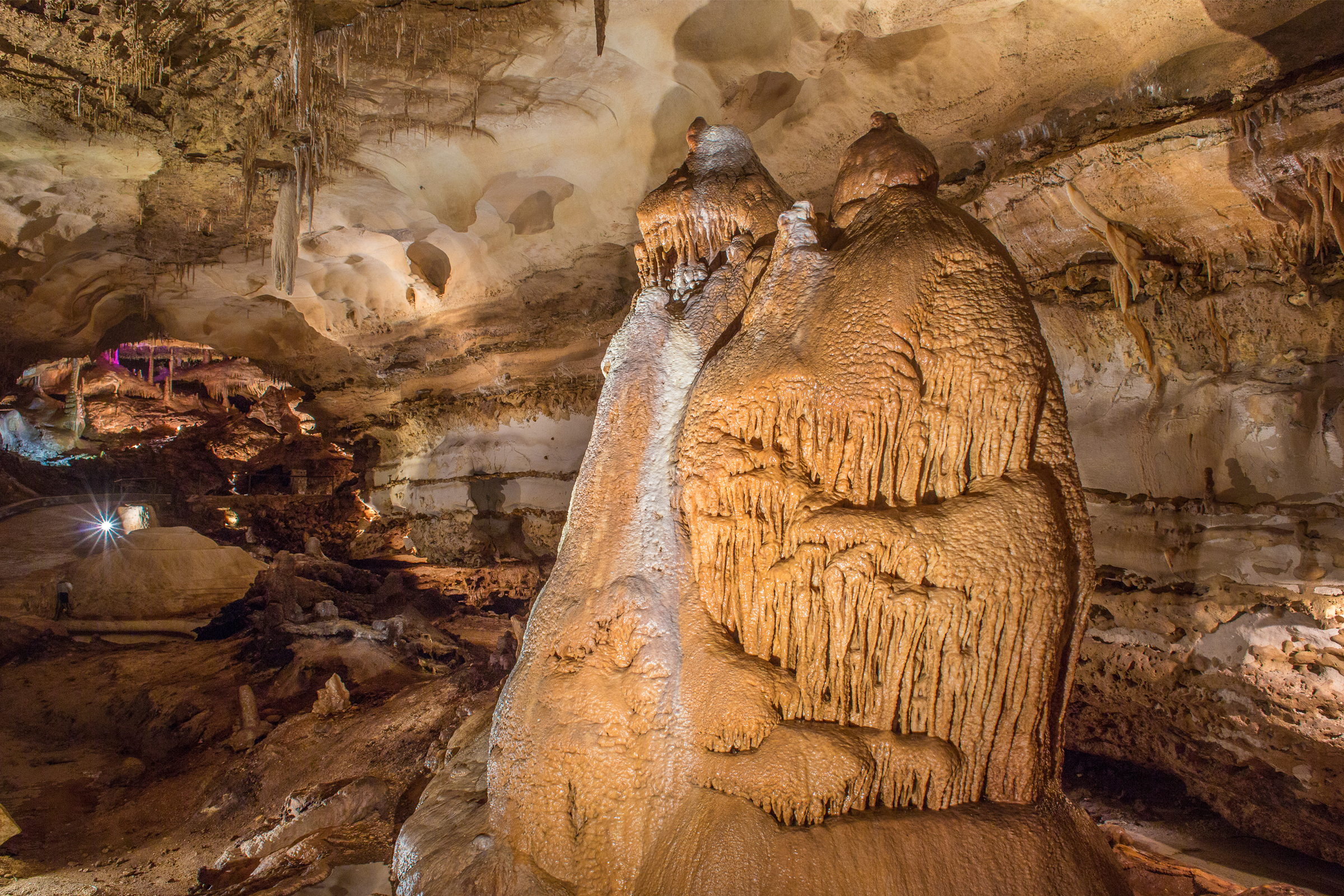This photograph captures the stunning interior of a well-lit cave, revealing its intricate natural features in sharp, vivid detail. Central to the image is a colossal stalagmite, ascending from the cave floor nearly to the ceiling, which strikingly resembles two human figures standing side by side or huddled together with sculptural precision. The formation, with its earth-toned, light mud color, appears almost like dripping stone, with one figure seemingly draped in a fringed shawl, underlined by an orangish-yellow hue and streaks of white cascading down its center due to the lighting.

The surrounding cave walls and ceiling display a fascinating array of earthy colors, from golden sandy yellow to various shades of brown, marked with cream and tan striations and bare sections. The layers of the rock formations showcase the geological history of the cave. Small stalactites hanging from the ceiling add to the textural richness of the scene.

To the left of the central structure, a gleaming spot suggestive of sunlight or artificial lighting enhances the natural beauty, casting intriguing shadows and light across the formations. In the distant background, the cave extends further, with additional stalactites, stalagmites, and crystal elements visible, hinting at the vastness and complexity of this underground wonder.